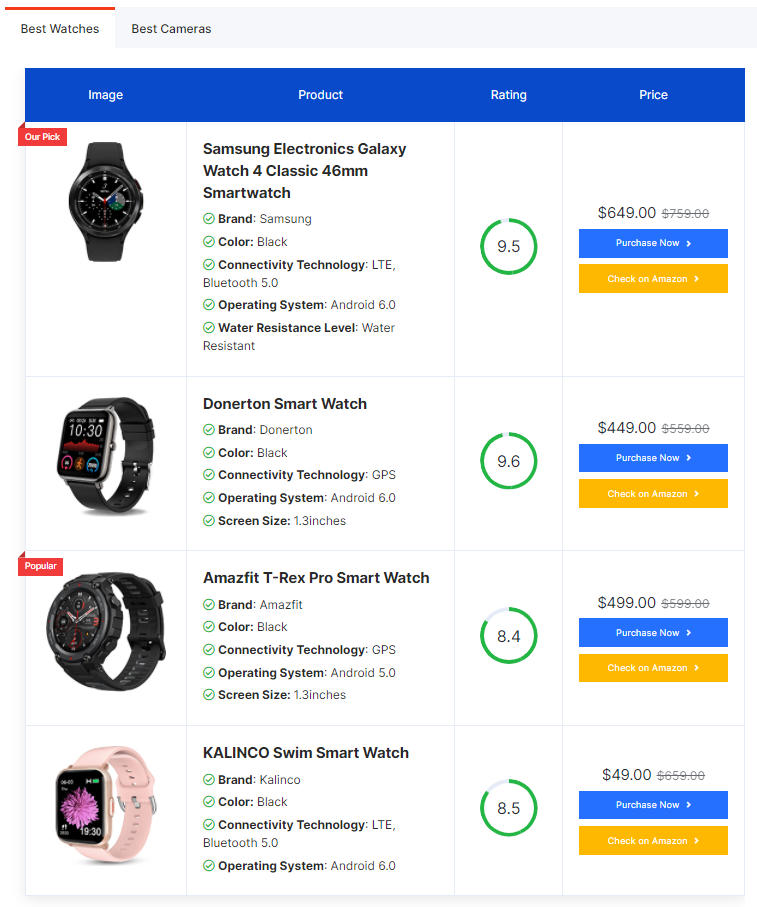This image is a screenshot showcasing a detailed comparison of top-rated watches, organized into several columns. At the top, the columns span downwards with distinct categories: the first column features images of the watches, the second column provides product information, the third column lists their ratings, and the final column displays their prices.

1. **Samsung Electronics Galaxy Watch 4 Classic (46mm)**:
   - **Image**: Black wristwatch
   - **Product Information**: Comprehensive details about the watch
   - **Rating**: 9.5
   - **Price**: $649

2. **Donerton Smartwatch**:
   - **Image**: Picture located on the left with accompanying information beneath
   - **Rating**: 9.6
   - **Price**: $449

3. **Amazfit T-Rex Pro Smartwatch**:
   - **Rating**: 8.4

4. **Kalinko Swim Smartwatch**:
   - **Rating**: 8.5
   - **Price**: $49

The product descriptions and ratings for the Amazfit T-Rex Pro and Kalinko Swim smartwatches are similarly formatted, though the exact prices and specific details beyond their ratings are not as thoroughly described in the provided text. This structured side-by-side layout allows for easy comparison of features, ratings, and prices among the top four smartwatch options.